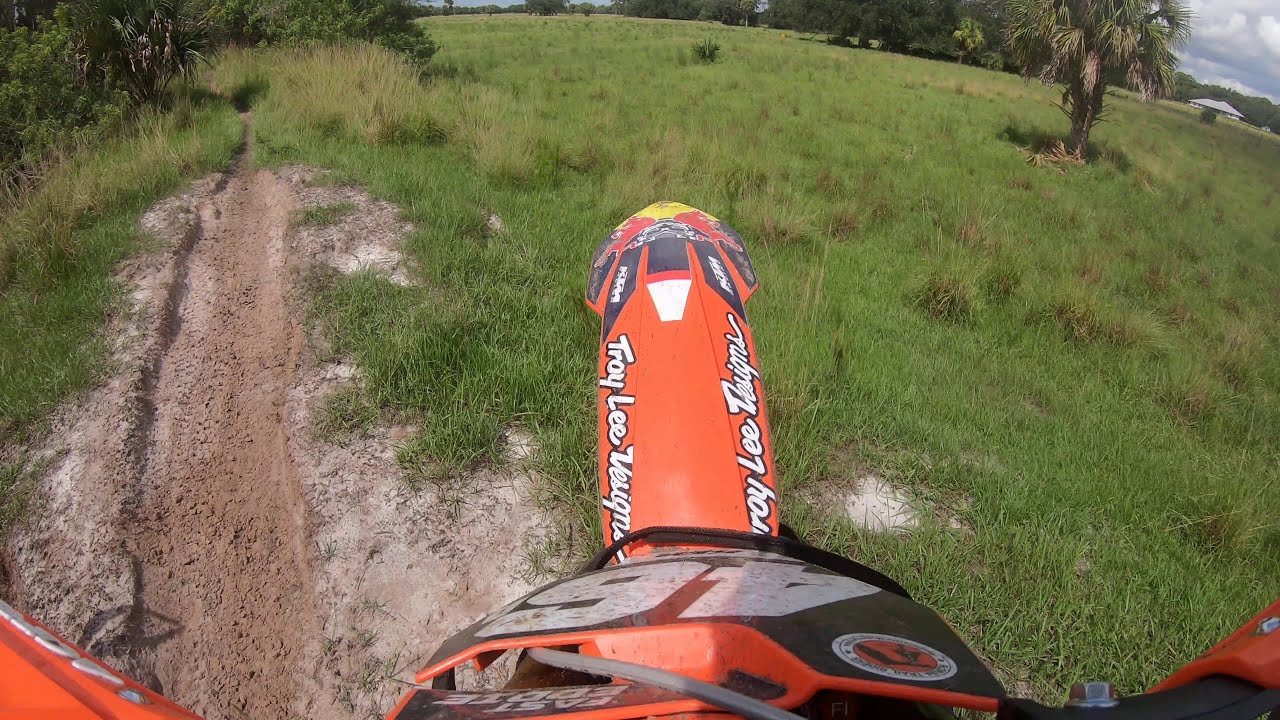This image, captured from the perspective of riding on a dirt bike, showcases the vehicle's prominent orange, black, and white color scheme, including an orange shield on the front tire and the digits "46" displayed near the handlebars. The scene is set in a grassy field dotted with dirt patches and a ditch-like area, likely an artificial dirt bike trail. The photo, taken during the daytime under a clear blue sky with light white clouds, also features a palm tree on the right side and multiple trees and bushes to the left. In the distant horizon, a dense line of trees stretches across the view. Additionally, a gray house can be spotted far off to the right. The foreground primarily consists of thick grass and occasional patches of dirt, adding to the dynamic outdoor setting.